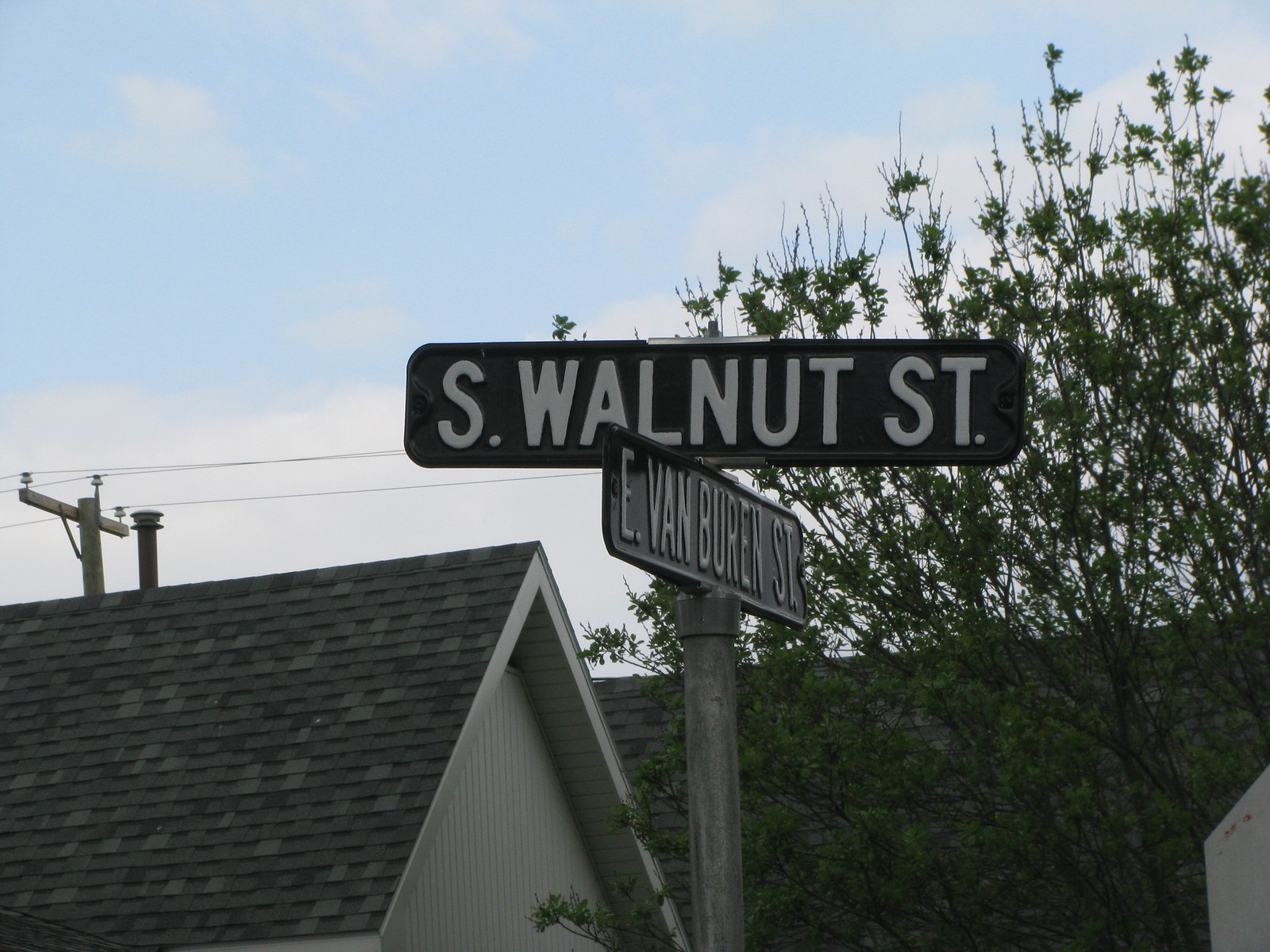This outdoor photograph captures a quaint residential intersection bathed in natural light on a semi-clear day. At the forefront, two black and white street signs affixed to a metal pole demarcate the cross streets of South Walnut Street and East Van Buren Street. The top sign prominently displays "South Walnut Street," while the bottom sign reads "East Van Buren Street." Above, the sky stretches out in a blend of blue and scattered white clouds.

Flanking the intersection, the image reveals the rooftops of two houses. On the right, partially obscured by a tree with slim branches, the lower roof showcases dark shingles and hints of the house's gray exterior. To the left of the tree, an A-frame roof rises slightly higher, its black and gray shingles forming a striking contrast against the sky. Both houses are surrounded by power lines that crisscross the scene, adding an urban touch to the otherwise serene neighborhood setting.